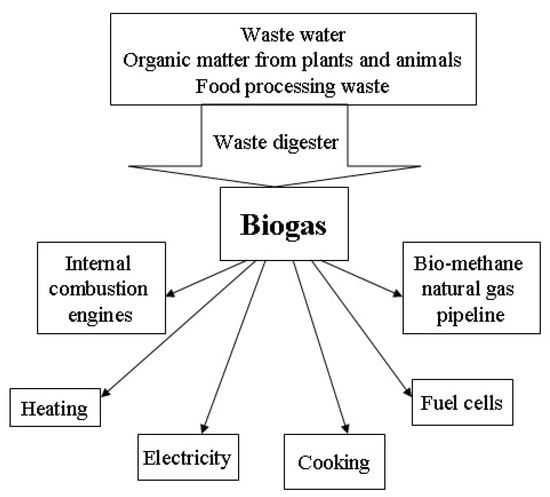The image is an infographic with a white background and black text, illustrating a process flow chart. At the top, a large rectangle contains the text: "Wastewater, organic matter from plants and animals, food processing waste." An arrow labeled "Waste Digester" points downwards to a smaller rectangle labeled "Biogas." From the biogas rectangle, six arrows fan out in a semicircle leading to six smaller rectangles, each representing a different application for biogas. These are labeled, from left to right: "Internal Combustion Engines," "Heating," "Electricity," "Cooking," "Fuel Cells," and "Biomethane Natural Gas Pipeline." This diagram outlines how waste materials are processed into biogas, which can then be utilized for various energy applications.